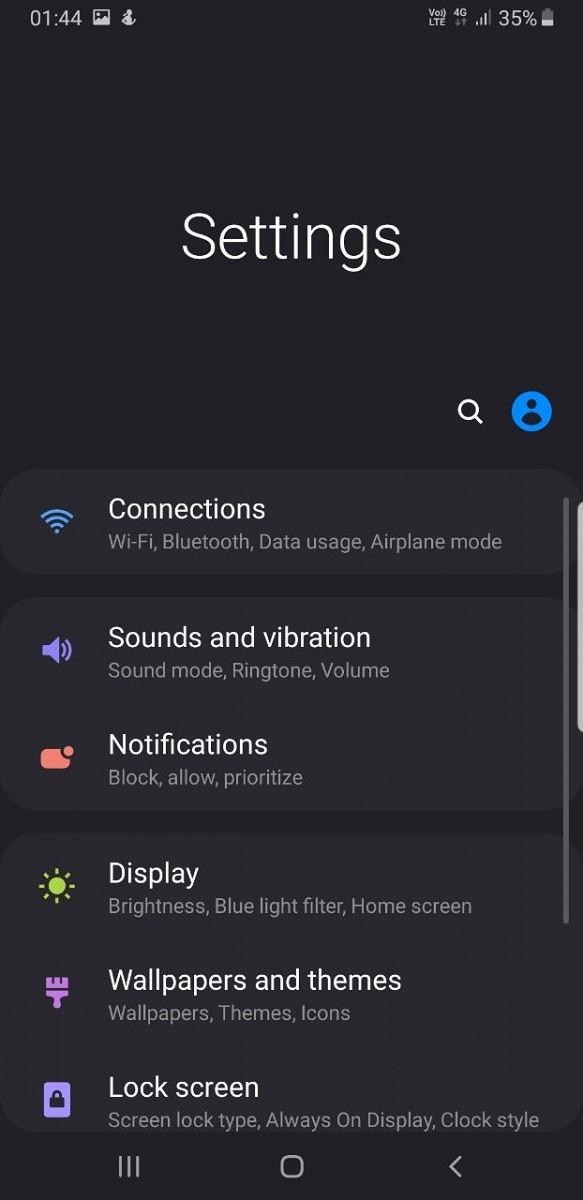The image showcases a screenshot of a smartphone's settings menu. At the top center, the title "Settings" is prominently displayed. To its right, there is a search bar icon and a blue circle featuring a standard profile icon. The menu is divided into several sections with various options:

1. **Connections:** Includes Wi-Fi, Bluetooth, Data Usage, and Airplane Mode.
2. **Sounds and Vibration:** Covers Sound Mode, Ringtone, Volume, and Notifications settings, with options to block, allow, or prioritize notifications.
3. **Display:** Manages settings for Brightness, Blue Light Filter, Home Screen, Wallpapers and Themes, with sub-options for Wallpapers, Themes, and Icons.
4. **Lock Screen:** Contains settings for Screen Lock Type, Always On Display, and Clock Style.

A gray scroll bar is positioned on the right side of the screen for additional navigation. At the very bottom of the display, there are three navigation buttons: a triple-line icon on the far left, a home button in the center, and a back arrow on the far right. The time shown is 1:44, and the battery level is at 35%.